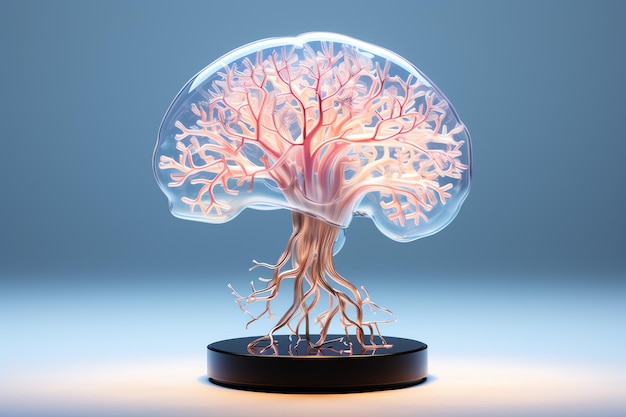The image features a perplexing and somewhat unsettling scene dominated by a structure resembling a tree or brain. The backdrop transitions from a darker blue at the top to a lighter blue-gray at the bottom, suggesting depth. The main object is an intricate, clear plastic or glass bubble encompassing an array of white and pink, vein-like branches. These branches emanate from the central mass, which distinctly mirrors the appearance of a brain with its complex network of nerve endings. The base of this peculiar structure is a solid, round, black platform. Supporting the brain-like mass are numerous root-like protrusions, which are a mix of white and brown hues, extending and intertwining around the base. The overall composition combines elements that evoke both organic and synthetic visuals, integrating a tree-like trunk and branching system with an anatomical brain structure, set against a softly graduated sky-blue background.